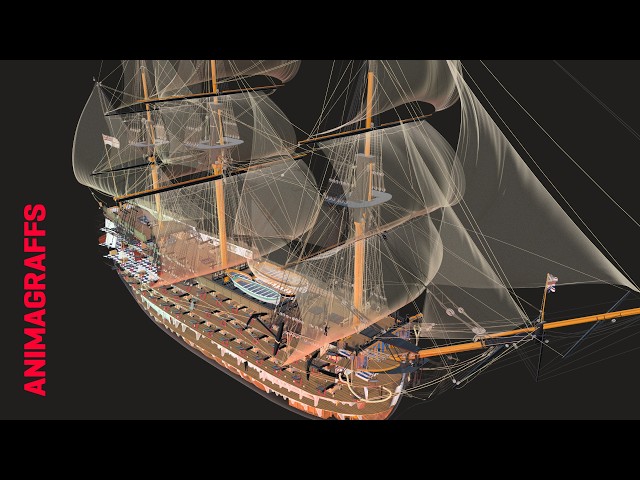This detailed illustration, entitled "How an 18th Century Sailing Warship Works" by Anima Graffs, serves as a YouTube thumbnail from the company. Dominating 75% of the image is a colossal 18th century warship, depicted with its many sails and intricate rigging. The diagram showcases the ship's interior with a cutaway view, revealing four distinct floors, each with a checkered pattern on the lower levels and a wooden floor on the top deck. The ship's upper structure features black and yellow coloring, with cannons protruding from its sides. In the foreground, a small figure stands at the bow, adding a sense of scale to the massive vessel. The scene is set against a light ocean backdrop with a creamy, foggy overlay blending into the sky. The title text is prominently displayed on the right, and a red text reading "Anima Graffs" is oriented vertically in the top right corner. Black borders frame the top and bottom of the image, completing the detailed and informative visualization of the historic warship's inner workings.